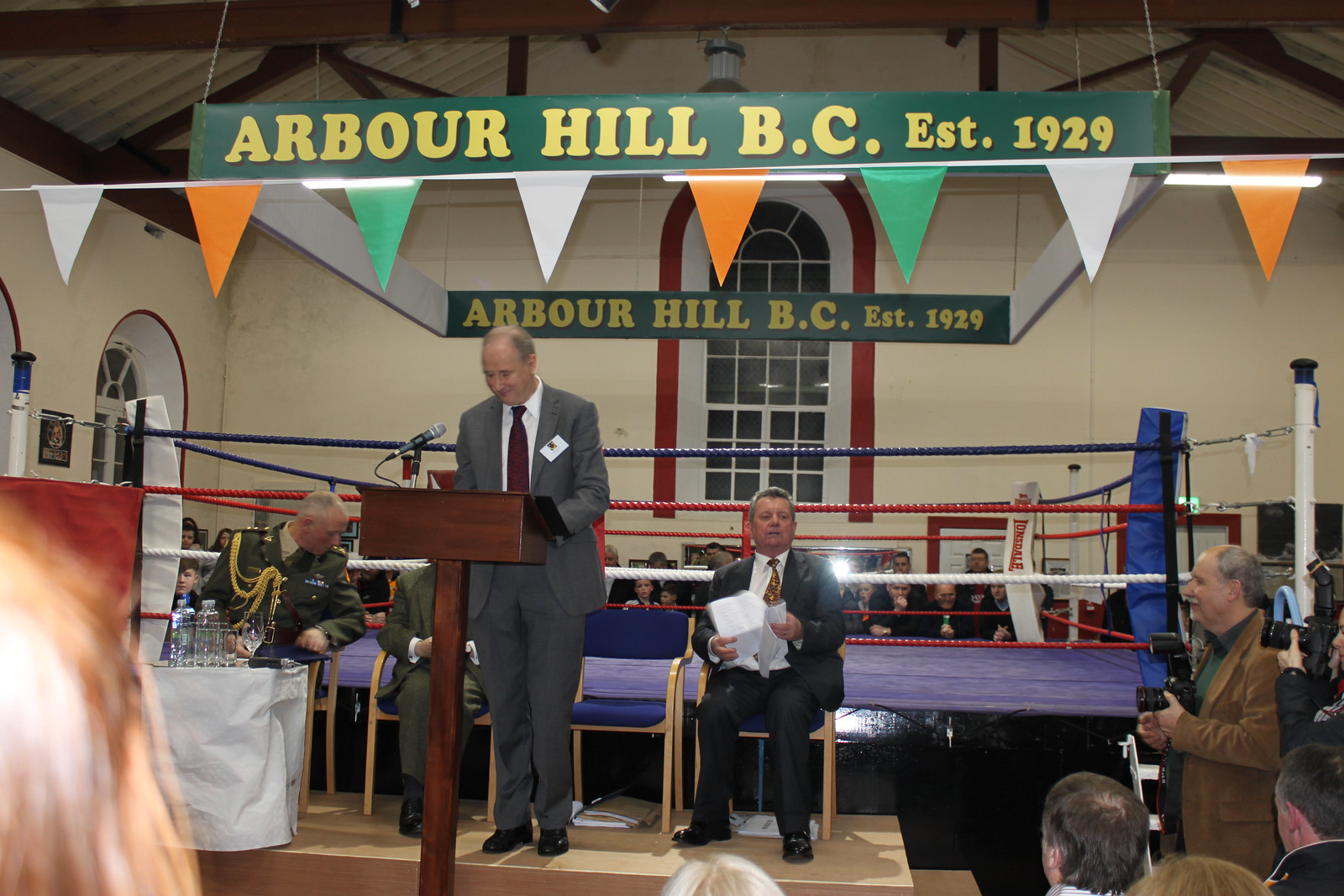In this detailed indoor photograph, three individuals are prominently featured on a stage in front of a blue boxing ring adorned with red, white, and blue ropes. Central to the image is a man in a medium gray suit with a maroon tie, standing at a brown wooden podium equipped with a microphone. To his left sits a man in military fatigues, identified by his decorated uniform, including an olive blazer and a golden rope decoration, sitting at a white table with water bottles. On his right is another man in a dark suit, seated on a wooden chair with blue cushions. The stage is set against a backdrop that includes a large, rounded window with red and white trim, and a banner overhead reading "Arbor Hill, B.C., Established 1929." The audience is visible both behind the ring and at the bottom of the photograph, with photographers positioned in the bottom right corner.